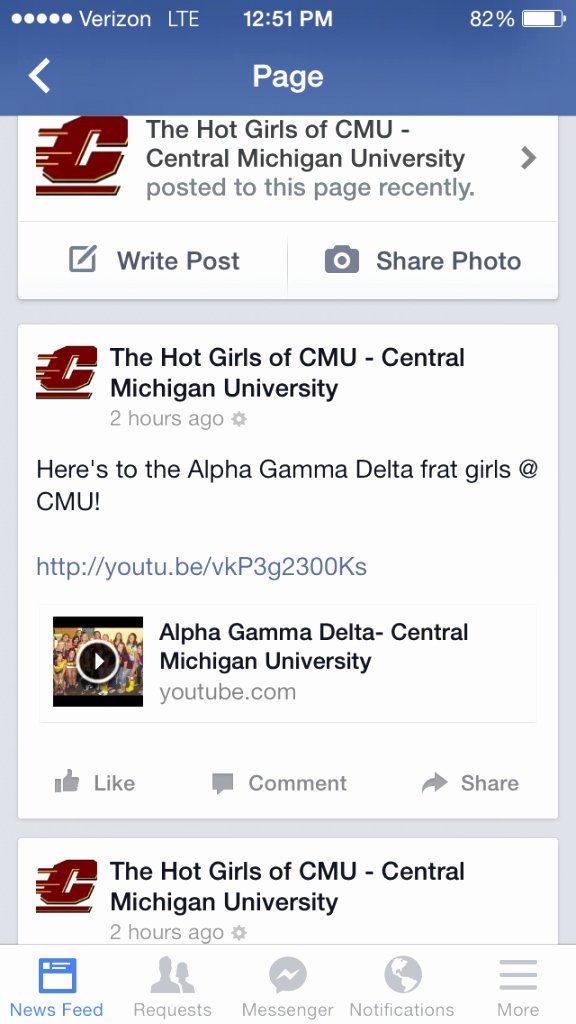Screenshot of a mobile phone screen displaying a social media page. At the top, a blue status bar indicates "Verizon LTE" on the left, "12:51 p.m." in the center, and "82%" battery with a battery icon on the right. Below the status bar, an interface section labeled "Page" features a back arrow on the left. The screen background is light gray, overlaid with white content boxes containing various information.

The top box features a circular "C" logo and reads, "The Hot Girls of CMU (Central Michigan University) posted to this page recently: Write Post or Share Photo." The following box, with the same logo, states, "The Hot Girls of CMU Central Michigan University, 2 hours ago. Here's to the Alpha Gamma Delta frat girls at CMU," followed by a YouTube link with the thumbnail and text: "Alpha Gamma Delta, Central Michigan University - YouTube.com."

Below the post are options to "Like," "Comment," and "Share." Another post from "The Hot Girls of CMU Central Michigan University" from two hours ago is partially visible. At the bottom of the screen, navigation buttons read "News Feed," "Requests," "Messenger," "Notifications," and "More."